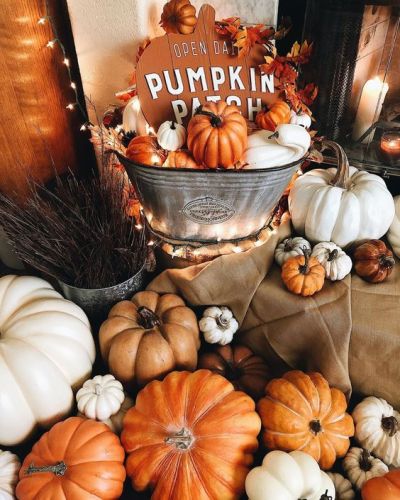The image showcases a festive storefront promoting a pumpkin patch, adorned with an array of autumn-themed decorations. Central to the scene is an orange, pumpkin-shaped sign with white text that reads "Open Daily" and "Pumpkin Patch" in larger font below. This eye-catching sign is nestled in a large steel bowl filled with an assortment of small, decorative pumpkins in shades of orange, white, and various other colors, likely artificial. The bowl is further embellished with a garland of multicolored autumn leaves in hues of brown and orange, and a string of white lights reminiscent of Christmas decorations, adding a warm glow to the display.

Behind this striking centerpiece, a white wall provides a neutral backdrop, ensuring the sign stands out. Below the steel bowl, the ground is scattered with a diverse collection of pumpkins ranging from large, typical sizes to smaller ones that fit in the palm of a hand. These real pumpkins come in a spectrum of colors including orange, brown, and white. Together, this charming and vibrant arrangement not only celebrates the season but also effectively invites passersby to visit the pumpkin patch.